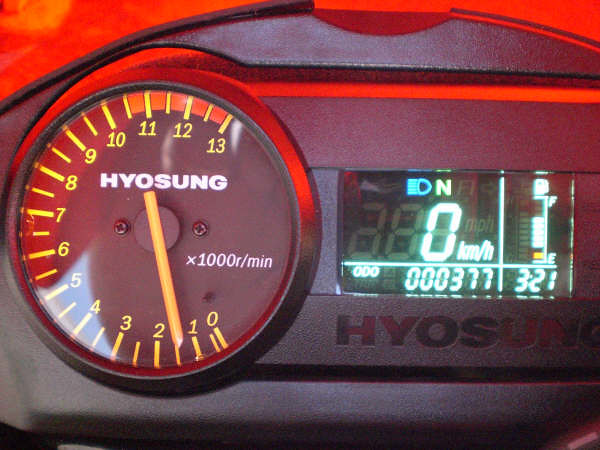This image showcases a close-up view of a meter panel, likely from a vehicle, branded with the HYOSUNG logo. The logo is partially visible in the bottom-right corner and fully displayed on the left side of the panel. The main circular gauge prominently features numbers ranging from 0 to 13, with a needle currently positioned between 1 and 2. Above this gauge, white text reads "x1000 R/min," indicating revolutions per minute.

Adjacent to the central gauge, a small rectangular digital screen displays "0 KM/H" and a fuel gauge marked with "E" for empty at the bottom and "F" for full at the top. The digital readout below shows the odometer reading "000377" with "321" beside it. At the top of the image, part of a red vehicle frame is visible, providing context to the meter’s placement.